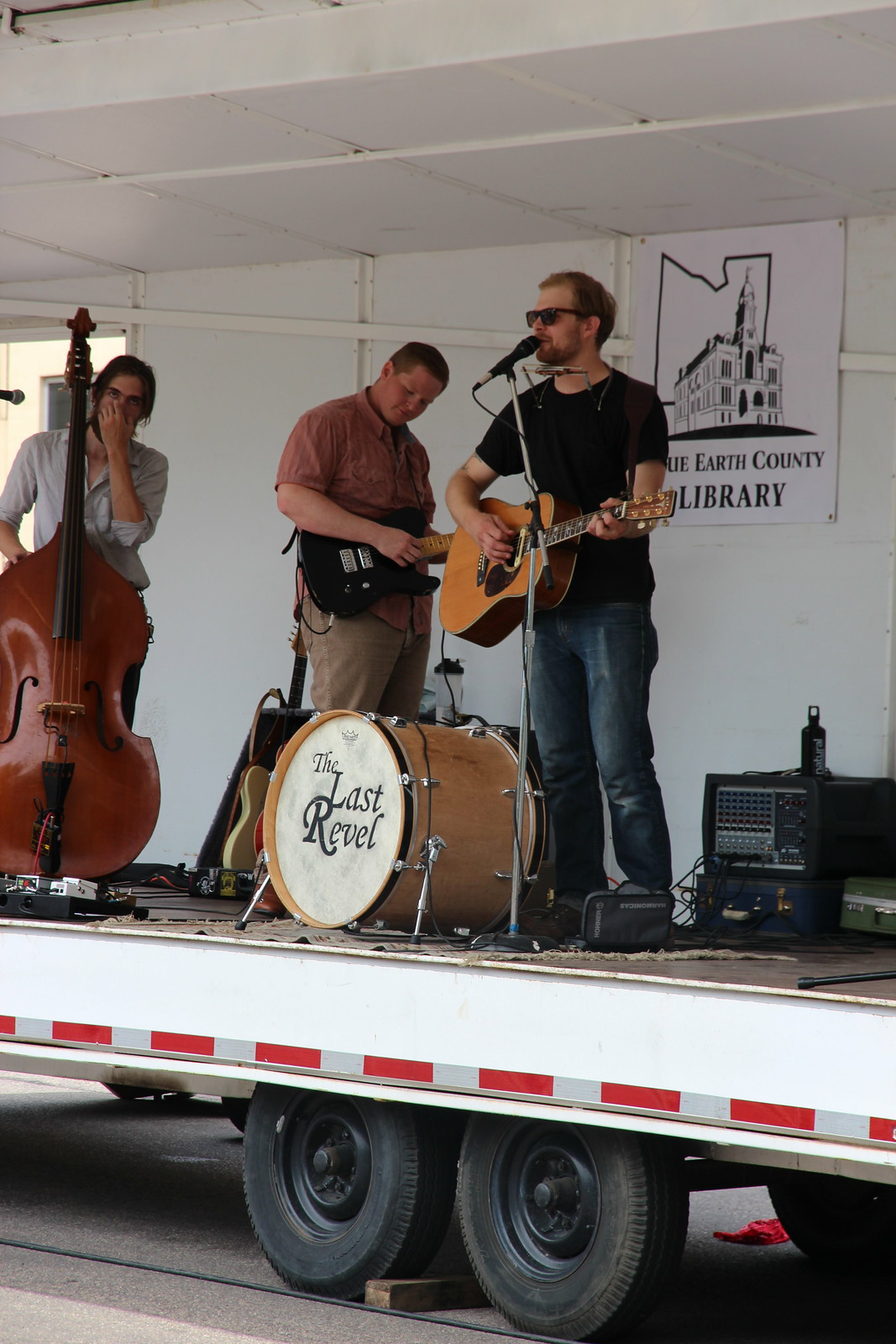The image depicts a trio of musicians performing on a stage that is part of a trailer, which has a white base with two visible black wheels underneath. The backdrop features a sign that reads "Earth County Library," and an illustration of an old building with a tower and an outline of an unidentified state. The band, named "The Last Revel," is composed of three members. 

On the far left stands a man with long hair, wearing a white collared shirt, playing an upright bass, which is a large wooden stand-up instrument nearly as tall as he is. At the center of the stage, a musician with a black t-shirt, jeans, short hair, light beard, and sunglasses holds an acoustic guitar and sings into a microphone. Positioned right in front of him is a bass drum with "The Last Revel" inscribed on its face. To the right, a third musician, dressed in khakis and a maroon collared shirt, plays an electric guitar with a black body. The trailer stage is entirely white within and fitted with some amplification equipment at the corner. The photograph captures these three musicians fully engaged in their performance, although no audience is visible.